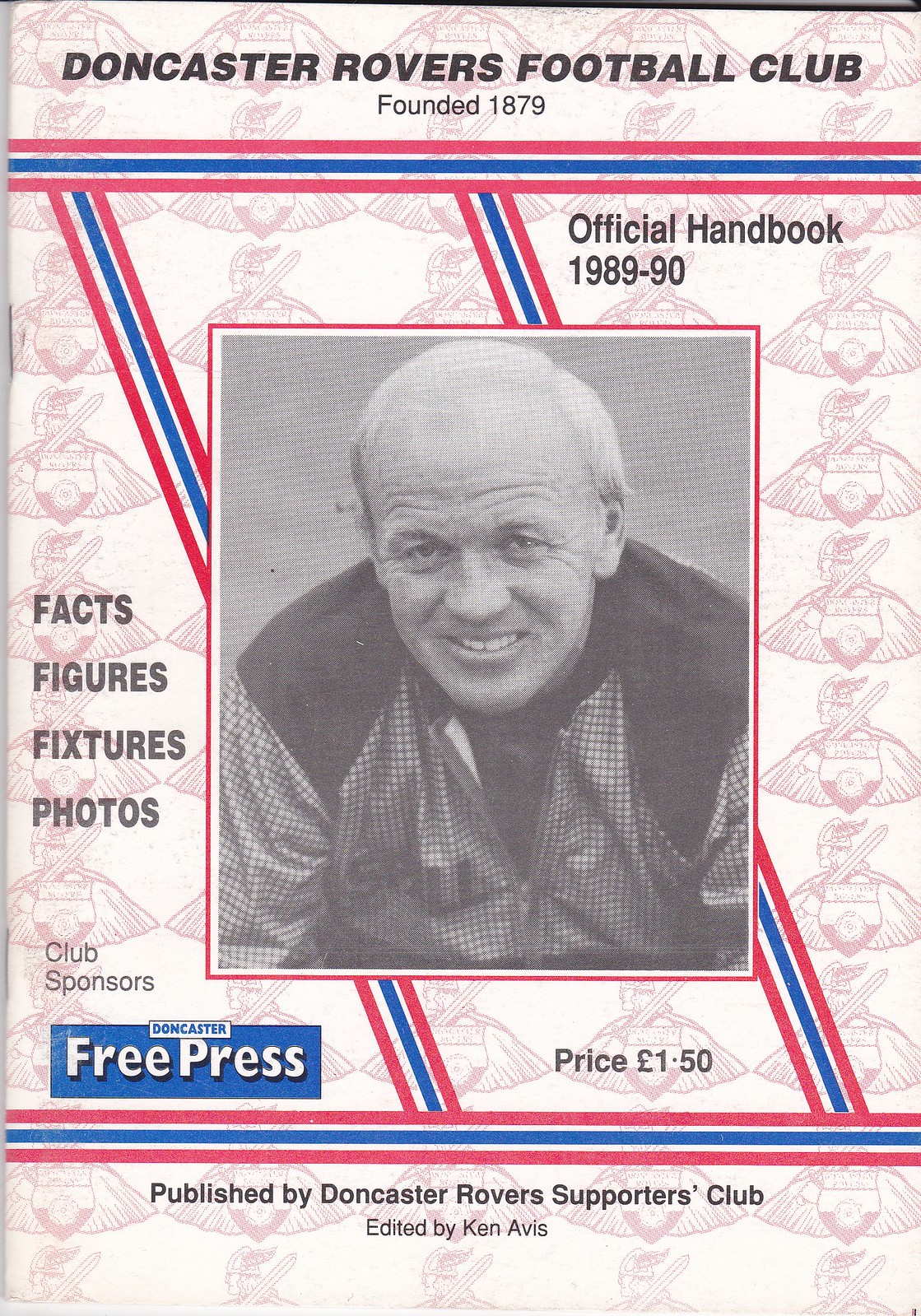This vertically oriented, rectangular image is the cover of a vintage booklet. The worn cover, slightly discolored to a light pinkish hue, is held together by two staples along the spine, one at the top and one at the bottom. The background features a repeating pattern of a Viking, depicted in a sideways view, holding a sword on his shoulder and a shield in front.

The header prominently displays "DONCASTER ROVERS FOOTBALL CLUB" in bold black uppercase letters, accompanied by the founding year, "FOUNDED 1879". Below this, three horizontal stripes (red, blue, and red) traverse the cover from left to right. Midway, "OFFICIAL HANDBOOK 1989-90" is printed in black on the right side. An interconnected set of diagonal stripes, identical in color, extends across the booklet from two points, segmenting the cover into distinct areas.

At the center, a black-and-white photograph of an older man with a bald top and grayish hair at the sides is framed by a red border. The man, who appears to be smiling, is dressed in a checkered shirt. To the left of his photograph, "FACTS, FIGURES, FIXTURES, AND PHOTOS" is emblazoned in bold black uppercase letters.

In the lower left, "CLUB SPONSORS, DONCASTER FREE PRESS" is noted, while the lower right corner simply lists "PRICE 150" (presumably £1.50). At the very bottom of the cover, additional text reads, "PUBLISHED BY DONCASTER ROVERS SUPPORTERS CLUB, EDITED BY KEN AVIS." Finally, a blue rectangular background at the bottom features the words "FREE PRESS".